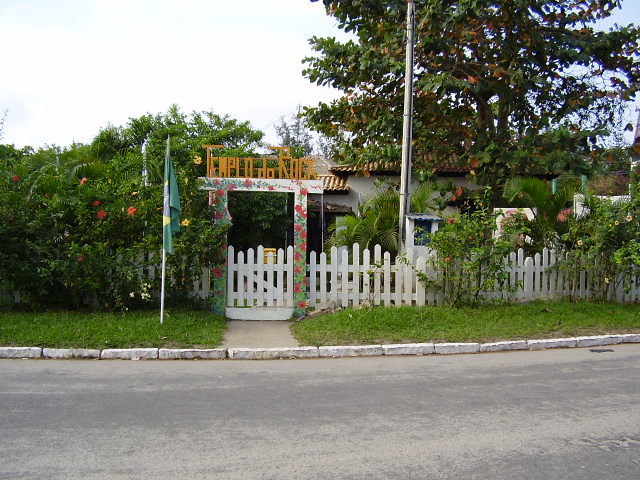The image depicts the entrance to "Templo do Rock," a rock and roll museum established by Brazilian rock legend Sergei in Rio de Janeiro, Brazil. The focal point is an intricately transformed house adorned with adobe on the roof, surrounded by a white picket fence. A striking sign with raised letters reading "TEMPLO DO ROCK" is mounted atop a wooden frame at the entrance, signifying the entrance to this unique venue.

In front of the house is a well-kept yard featuring a grassy lawn and blooming rose bushes, some of which extend dramatically over the fence line. A small flag is staked into the ground near the entrance gate, adding to the picturesque scene. The street in the foreground is empty, lined with white stone pavers and a narrow grassy median. A towering tree stands majestically in the yard, extending high above the house. The overall setting, devoid of people and cars, evokes a serene atmosphere.